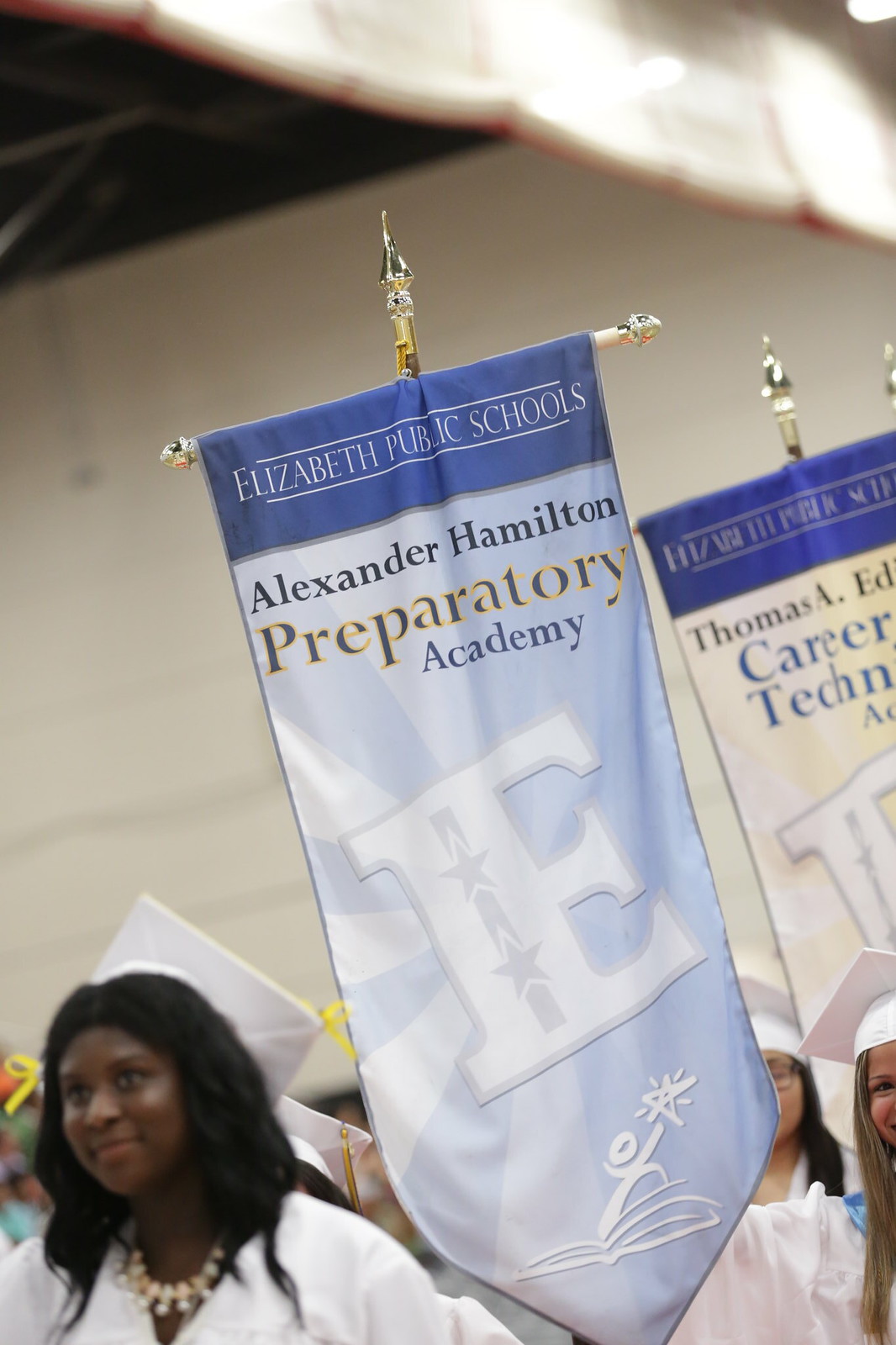The digital photograph captures a graduation ceremony at Elizabeth Public Schools, specifically from Alexander Hamilton Preparatory Academy. The image predominantly displays a group of young women, each dressed in white caps and gowns, symbolizing their accomplishment. Prominent in the scene are large vertical banners—especially notable is the one with a horizontal type staff and a vertical pointed gold staff at the top. This banner, set against a light blue background, features a large capital "E" diagonally centered on it and bears the text "Elizabeth Public Schools" within a blue rectangle at the top and "Alexander Hamilton Preparatory Academy" below. Additionally, a banner for Thomas A. Edison Career Technologies is visible in the background. The setting may be a school gymnasium, brightly lit from the right side of the image. Behind the graduates, a mix of other people, likely family members, can be seen, enhancing the festive atmosphere. The colors white, gray, light blue, royal blue, gold, and yellow dominate the photograph, adding to the celebratory ambiance of the occasion.